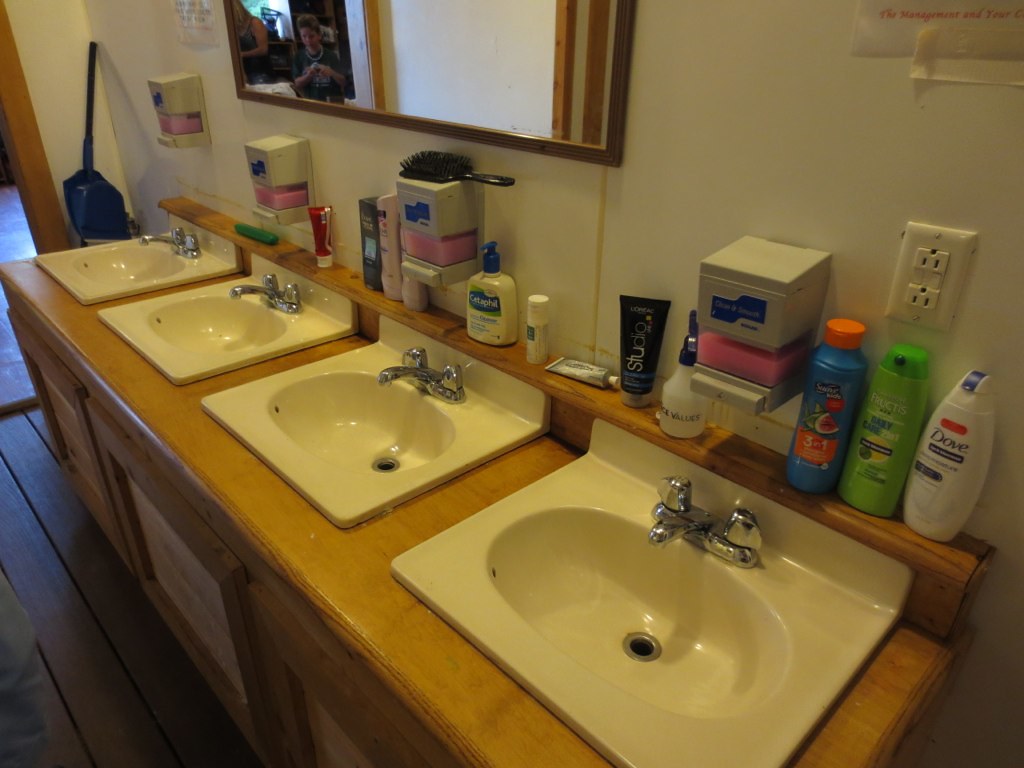The photograph features a row of four ceramic bathroom sinks with chrome faucets, all set in a light tan wood countertop that appears slightly slanted from the top left to the bottom right of the image. Above the sinks, there is a riser or backsplash lined with an array of hygiene supplies and toiletries. These include a white Dove bottle, a green Fructis bottle, a blue bottle with an orange cap, multiple soap dispensers containing pink soap, various toothpaste tubes, a Cetaphil pump bottle, and an assortment of other lotions and creams. Above this riser, a large vanity mirror reflects a person taking the photograph, as well as a partial view of a white wall. On the far left of the image, a blue broom and a dustpan are visible. The overall impression suggests a shared or communal bathroom, possibly in a dormitory or multi-family residence, due to the extensive lineup of grooming products and the practical layout of the sinks and counter space.